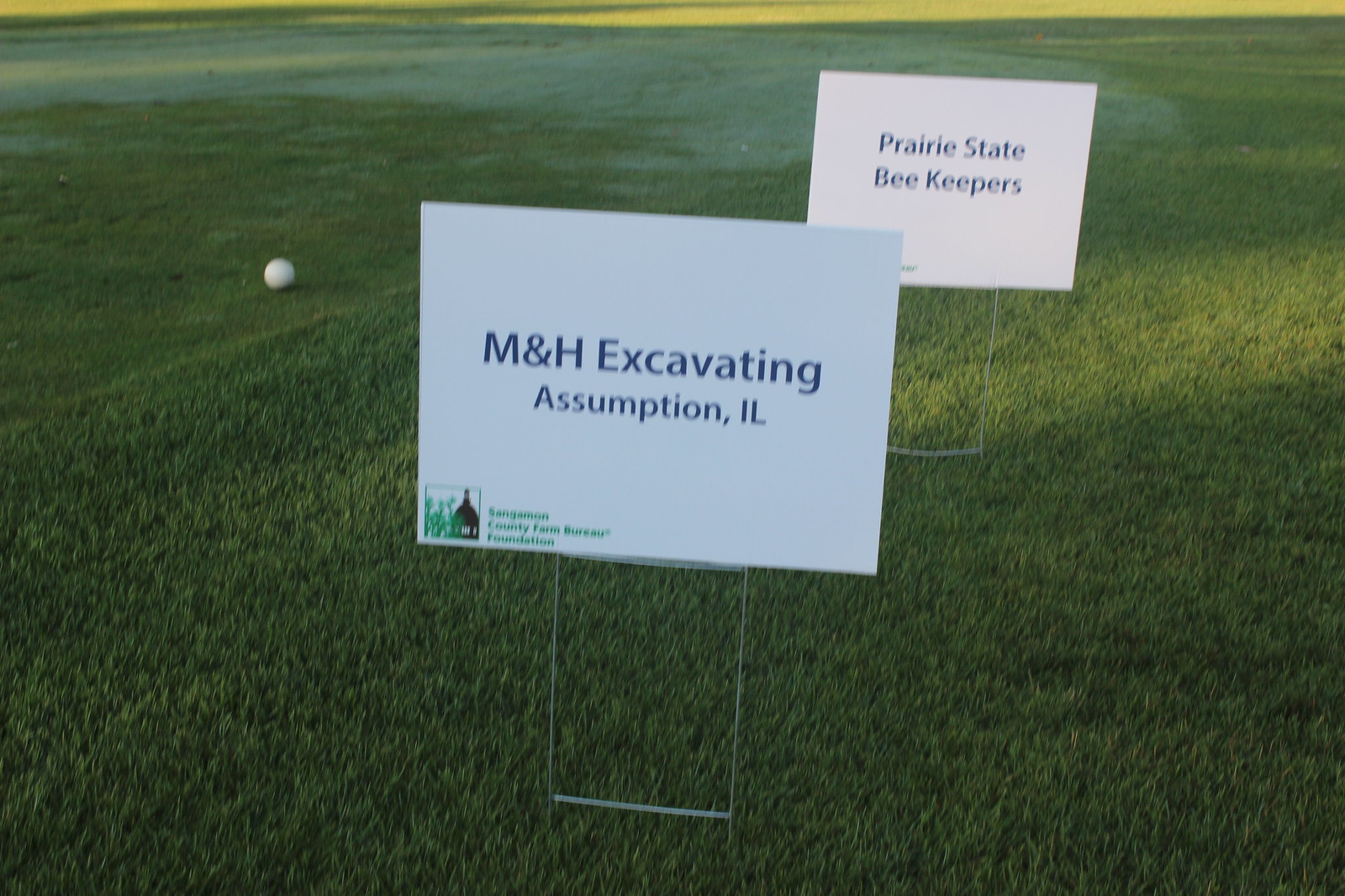The photograph captures a scene on a golf course with a mix of sunlit and shadowed greens, featuring a combination of longer grass in the foreground and shorter, manicured grass to the left. Prominently displayed in the image are two white yard signs with dark navy blue text, positioned on wire bases. The sign in the foreground reads "MNH Excavating, Assumption, IL," accompanied by a small logo at the bottom left that mentions "Sagamon County Farm Bureau Foundation" in green. Partially obscured by the first sign, the second sign reads "Prairie State Beekeepers." A golf ball is visible on the fairway to the left of the signs. In the background, there is a patch of bluish-green grass, completing the verdant landscape.